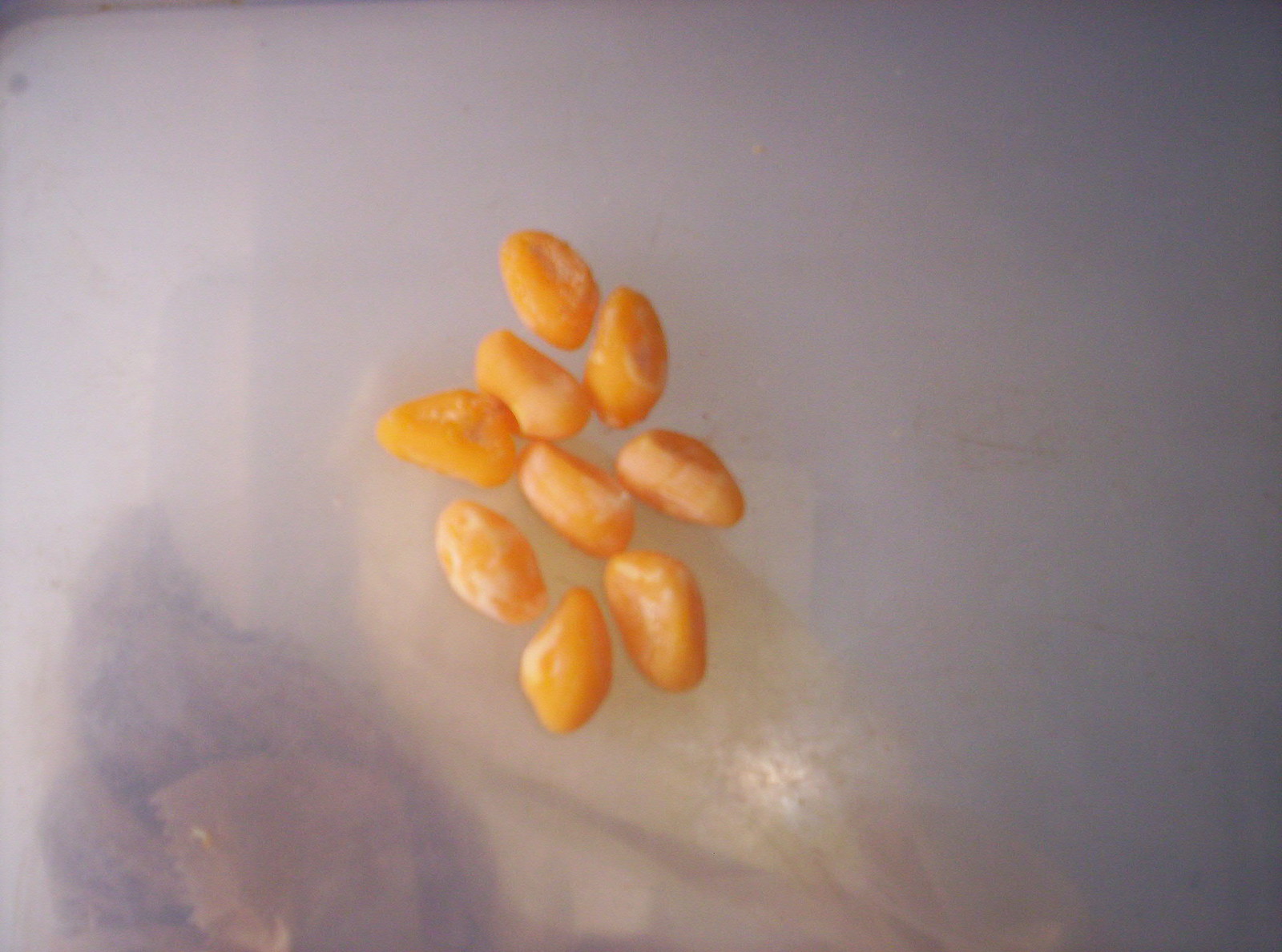This image features nine uniformly yellow-orange, oblong-shaped objects resembling seeds or small candies, reminiscent of sugar babies or mini mangoes. These objects display a subtle white haze or cast on parts of their surfaces. Arranged centrally on an opaque white, likely semi-translucent background, the setting appears partially cloudy or foggy. In the bottom left, there’s a reflection suggesting the presence of a darker, greyish-brown area with a lighter, off-white slanted rock-like form. The objects seem suspended in this hazy environment, adding to the image's surreal quality.